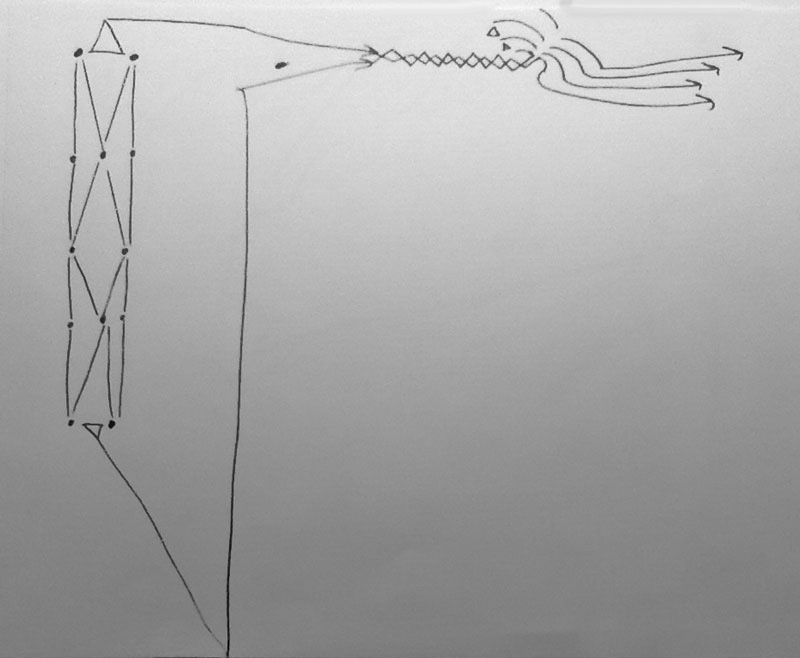This image features a sheet of paper showcasing an intricate pen drawing, predominantly positioned towards the left side of the sheet. Centrally, there is a long rectangular shape containing two prominent X formations. Each X is segmented by dots placed between the lines composing the structure.

Adjacent to the rectangular shape, additional dots create complex triangular and diamond shapes. At the top and bottom edges, there are individual triangles: the upper triangle points upwards, while the lower triangle points downwards. Each of these triangles has lines extending outward. 

From the upper triangle, a line projects to the right, terminating at a point with a dot. This configuration forms another triangle. From this second triangle, a line continues downward, creating a secondary triangular shape that connects back to the original triangle to the left.

Extending from the peak of the topmost triangle is a diamond-like design featuring a chain-link pattern. This design incorporates lines that culminate in four arrows pointing towards the right side of the composition.